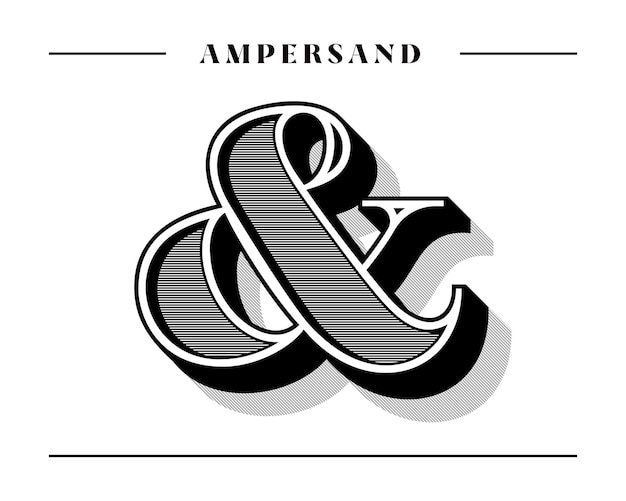The image is a computer-generated illustration of an ampersand symbol. At the very top of the image, the word "ampersand" is written in black text, surrounded by two short horizontal black lines—one to the left and one to the right. The illustration's background is white, and another horizontal line extends across the entire width at the bottom. 

At the center of the image is a large, bold, italicized ampersand symbol. The ampersand is depicted in a thick, 3D style with a white border outlined in black. Its interior appears hollow but is filled with intricate, tiny black strands, giving it a textured appearance. The ampersand's form features a flowing, curved shape, beginning at the top, looping down to the left, swinging back to the right, and ultimately resembling a 'J' shape at the bottom that curves back into the initial structure. The design also includes black 3D shadows and lighter grey shadows to enhance its three-dimensional effect, making the ampersand appear as though it pops out from the flat surface.